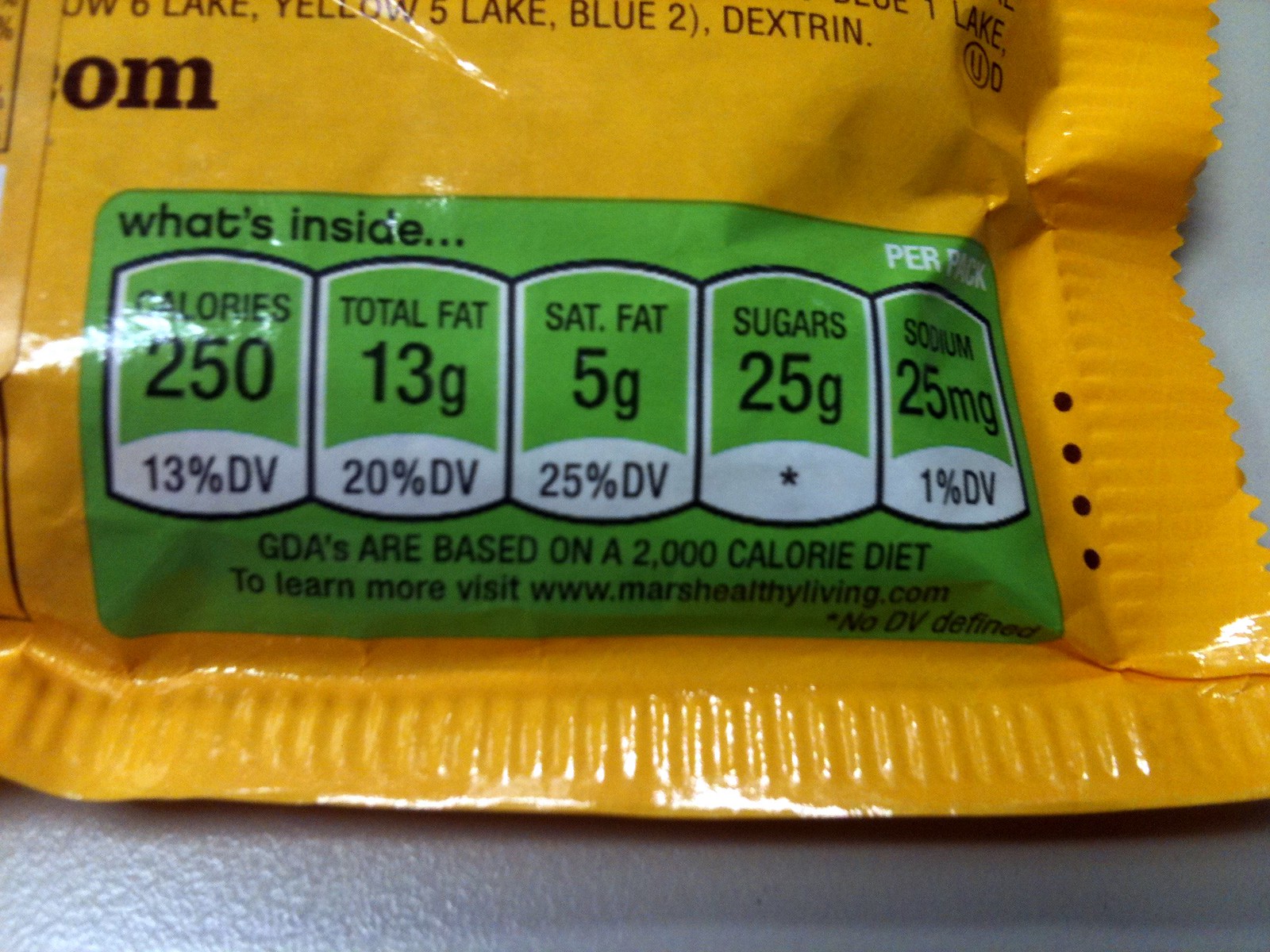This detailed close-up photograph showcases the nutrition facts label on a bag of M&Ms. The image highlights the "What's Inside" section prominently displayed in green, providing detailed nutritional information about the candy. The yellow packaging of M&Ms is visible in the background, creating a vibrant contrast that draws the viewer's attention to the green label. The label details that each pack contains 250 calories, 13 grams of total fat, 5 grams of saturated fat, 25 grams of sugars, and 25 milligrams of sodium. It notes that these values are calculated based on a 2,000 calorie daily diet, indicated by the GDA (Guideline Daily Amounts). There's also a web address, marshealthyliving.com, encouraging consumers to seek more information. The green color of the label appears to be a strategic choice, possibly implying a misleading sense of healthiness due to the common association of green with healthy products.